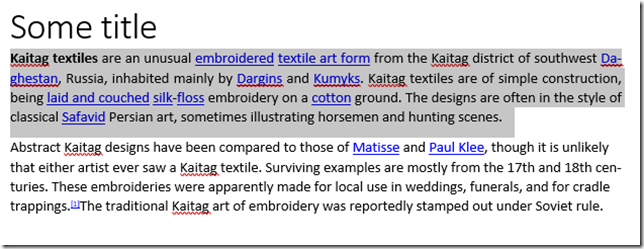The image features a block of text with a title in bold black letters, although the specific title is not provided. The main text describes Kaitag textiles, an unusual embroidered art form originating from the Kaitag district of Southwest Dagestan, Russia, an area primarily inhabited by the Dargins and Kumyks people. Kaitag textiles are characterized by their simple construction, utilizing laid and couched silk floss embroidery on a cotton ground. The designs often reflect classical Safavid Persian art styles, depicting scenes such as horsemen and hunting. Notably, abstract Kaitag designs have been compared to the works of Matisse and Paul Klee, although it is unlikely that these artists ever encountered a Kaitag textile. Most surviving examples date back to the 17th and 18th centuries and were made for local uses including weddings, funerals, and cradle trappings. The traditional art of Kaitag embroidery was reportedly suppressed under Soviet rule. The text includes highlighted words, akin to hyperlinks, for terms such as "embroidered textile form," "Dagestan," "Dargins," "Kumyks," "Safavid," "laid and couched silk floss," "cotton," "Matisse," and "Paul Klee." The lower part of the text discusses these textiles further but is not fully detailed in the provided content.